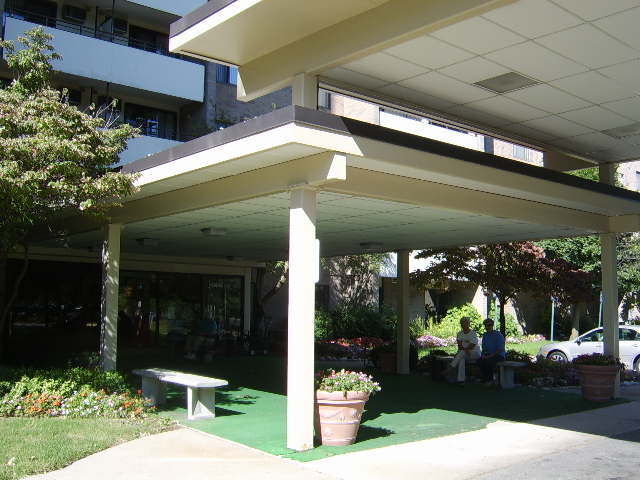This photograph captures the entrance of a large, white building, which could be a hotel, office complex, or possibly a golf club. The entrance features a substantial covered porch or patio area supported by white metal posts and topped with a white and black roof. This structure includes a ceiling that drops down inside, creating a sheltered space. A green artificial turf carpet mimicking grass covers the ground beneath the porch.

Two older women are seated on a gray stone bench positioned towards the left side of the covered area. The woman on the left wears a white top and white pants, while the woman on the right is dressed in a blue top and black pants. Opposite them, there is another gray stone bench. 

Surrounding the area are flower pots filled with vibrant flowers and well-maintained greenery, including bushes and trees situated to the left side of the porch. In the background, behind the women, a parking lot is visible with at least one car parked. Additionally, the area to the right of the porch serves as a carport where vehicles can drop off passengers. The building itself extends beyond the top of the image, indicating it has multiple levels. 

Sliding glass doors under the porch provide entry into the building, though they are partially obscured by the structure's pillars and awning.